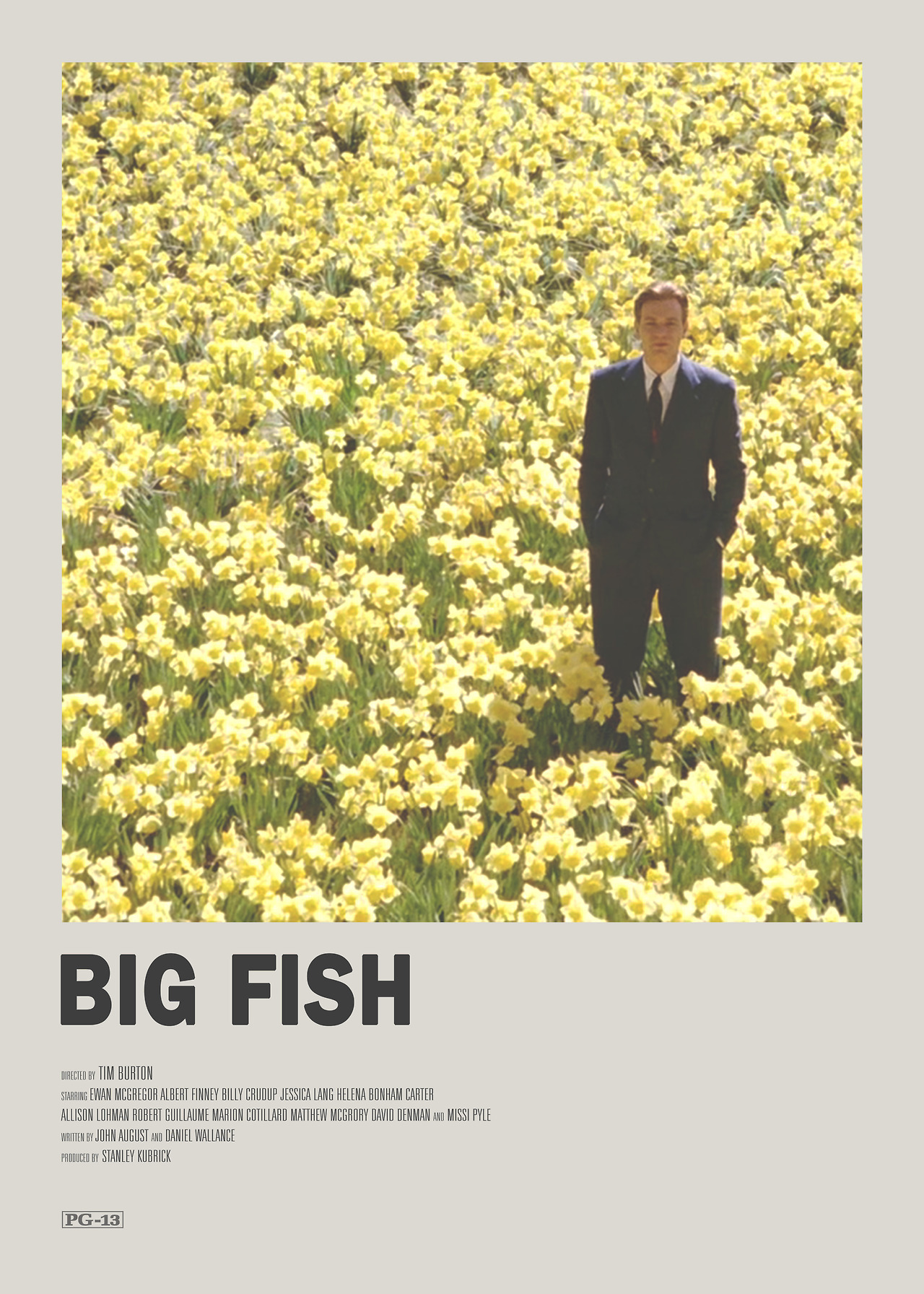The movie poster features a portrait-oriented design with a pale grayish background. Dominating the top two-thirds of the poster is a square image of a field filled with vibrant yellow daffodils, their green stems visible beneath them. In the midst of this field stands a man in the distance. He has short, blond hair and wears a blue suit with a dark tie, his hands casually placed in his pockets. The man looks directly at the viewer with a neutral expression. Below this central image, in large black capital letters, is the title "BIG FISH," followed by "directed by Tim Burton" in smaller print. Near the bottom, close to this text, is a listing of the starring actors, including Ewan McGregor, Albert Finney, Billy Crudup, Jessica Lange, and Helena Bonham Carter. In the bottom left corner of the poster, there is a small rectangle with the PG-13 rating.